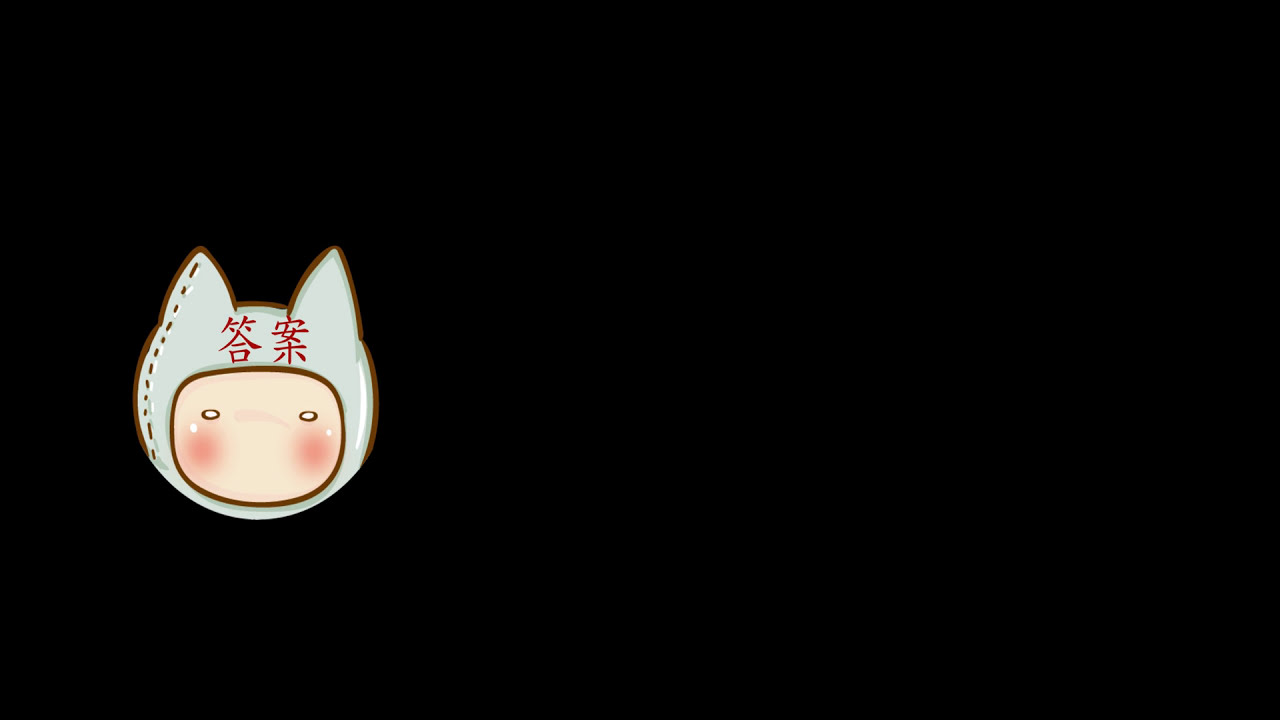The image is a simplistic graphic with a predominantly black, landscape-oriented background. Positioned in the middle of the left side is the focal point—a cartoony face wearing a distinctive hat. The face is a featureless, rounded rectangle with minimalist ovals for eyes, rosy cheeks adorned with small white dots, and devoid of a nose or mouth. This face, possibly resembling an anime character, is snugly enwrapped in a wraparound bunny or cat hat. The hat, in shades of gray, drapes beneath the chin and rises to form two short, pointy ears atop the head. Adding to the visual interest, two red Chinese or Japanese symbols are prominently displayed above what would be the forehead, and dashed lines along the hat suggest its soft, fabric nature.